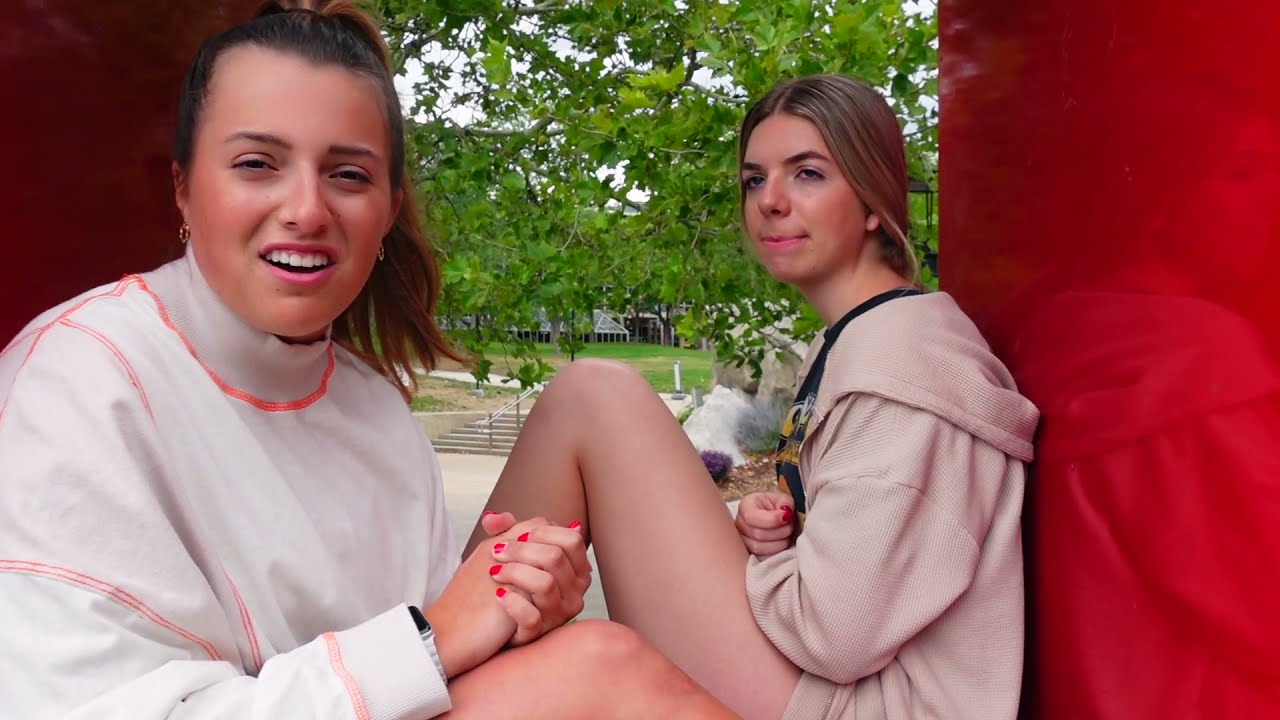In this outdoor photograph, two young women are sitting on what seems to be a building ledge, with green tree branches and leaves forming a lush backdrop. The image also captures a stair set and a sprawling grass field, hinting at a campus-like environment. Both women have their hair styled in ponytails and their nails painted red.

On the left, a girl with brown hair, wearing a white long-sleeved jacket with distinctive orange stitching, is smiling and appears to be engaged with the viewer. Her attire resembles a turtleneck. To her left rests a bag on a red reflective pillar.

On the right, the other girl is wearing a more pink-toned hoodie paired with short shorts and a black T-shirt. She has a contemplative expression, gazing slightly leftward. Her bag is similarly positioned on another red reflective pillar. Among the various colors in the photo, notable ones include white, pink, red, green, and earthy tones, accentuating the natural and serene atmosphere.